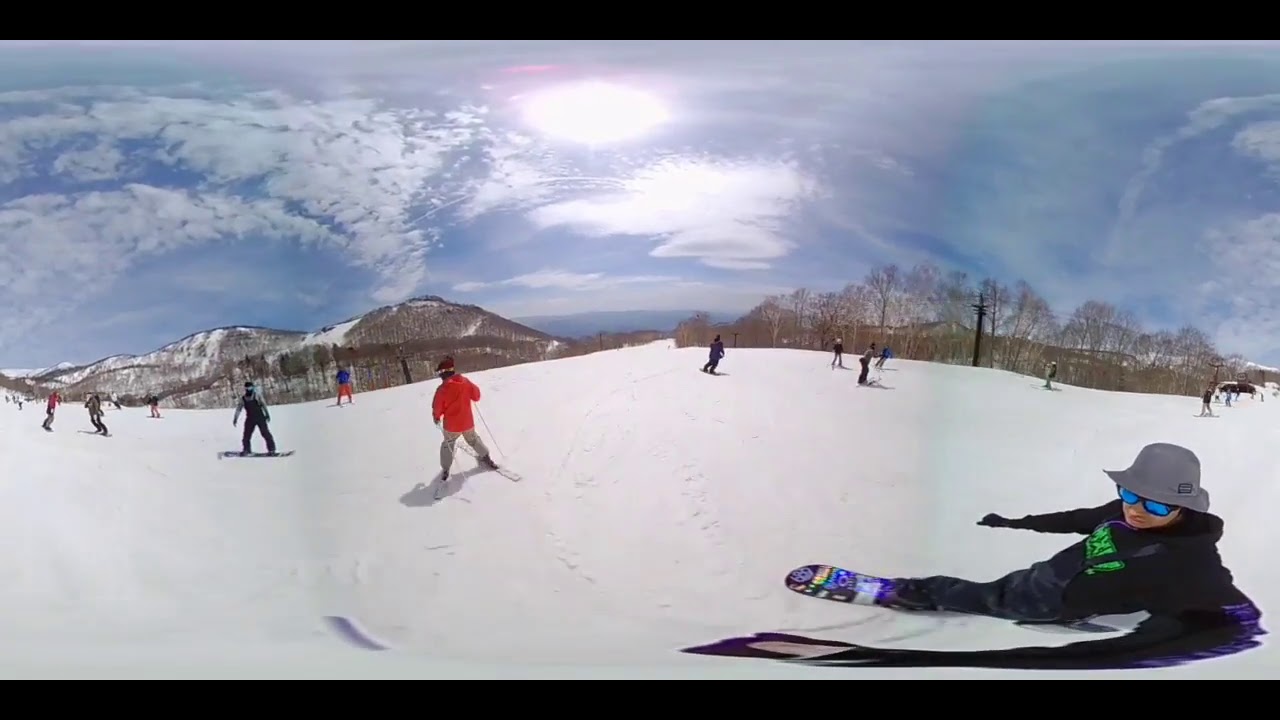A vibrant scene at a bustling ski resort, captured through a wide-angle lens, shows a diverse group of around 10 to 12 skiers and snowboarders amid scenic winter landscapes. In the foreground, a person in a black outfit with green goggles, black gloves, and a white hat stands on a decorated snowboard, taking a selfie with their phone. Just to the right bottom, another individual in a gray hat, blue sunglasses, and a parka with green lettering lies in the snow beside what looks like a snowboard. A red-jacketed skier and other enthusiasts in colorful gear navigate the slopes in various directions. Three visible trail options diverge from the same point indicated by the presence of ski poles and cables of a ski lift to the right, though the lift itself is not visible. The background is dominated by snow-covered mountains, with a tree line three-quarters up their slopes. The sky overhead is a beautiful mix of light blue and white, featuring irregular clouds, hints of sun, possibly a sun dog, and a touch of pink near the sun, painting a picturesque winter wonderland.